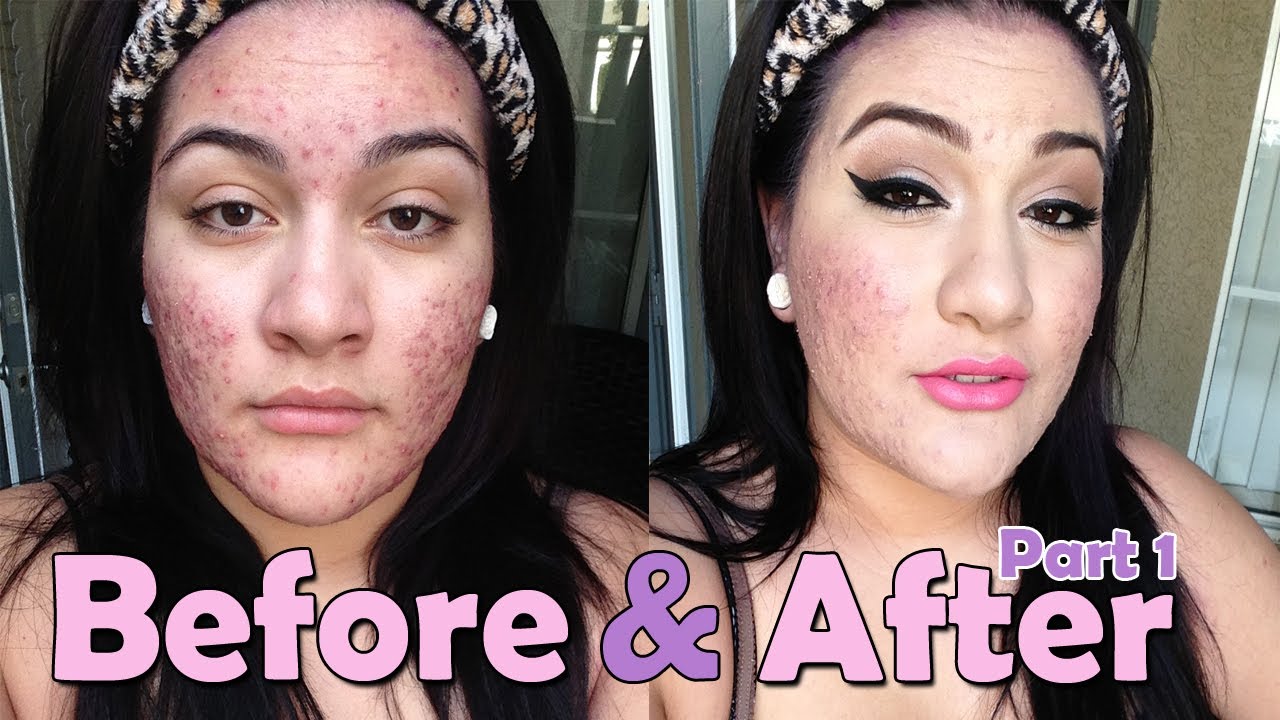The image is a side-by-side, before-and-after shot of a woman, likely depicting the effects of an acne treatment product in an advertisement. The photographs predominantly focus on the woman's face. She has long, dark hair, and in both images, she's wearing a leopard print headband. In the "before" photo on the left, her face shows acne on her cheeks, chin, and forehead. In contrast, the "after" photo on the right shows a significant reduction in acne, particularly on her forehead and chin, while some acne remains on her cheeks. Notably, in the "after" image, the woman is wearing makeup, including fishtail eyeliner and pink lipstick, whereas the "before" image shows her without makeup. The text overlay includes "Before" and "After" in pink, with the ampersand in dark pink. Above these words, in a smaller font and dark pink color, it reads "Part One." In the "after" photo, she appears to be outside, with a window visible in the background.